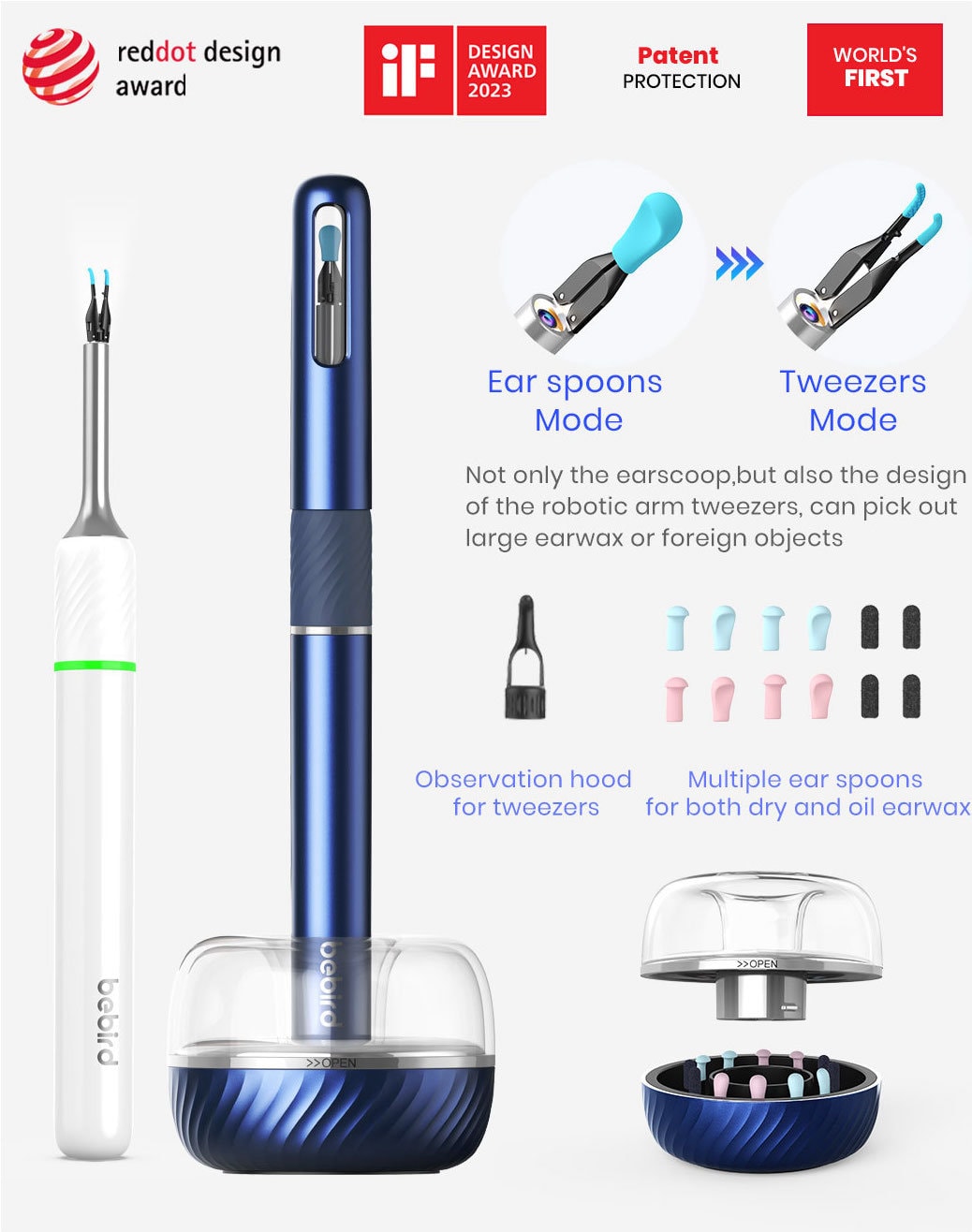This magazine page showcases a cutting-edge ear cleaning tool, honored with the Red Dot Design Award, Design Award 2023, and secured by Patent Protection, underlining its status as the world's first of its kind. Positioned in the top left corner is a ball with red and white stripes, bearing the Red Dot Design Award logo. The featured device boasts an innovative design, offering both "Ear Spoons Mode" and "Tweezer Mode". The sophisticated tool is engineered to effectively clean ears, using either ear spoons for dry and oily earwax or robotic arms tweezers for extracting large earwax or foreign objects. An Observation Hood for tweezers enhances precision. The device resembles a pen and includes a stand for easy storage. Equipped with a camera at its tip, it connects via Bluetooth, allowing users to watch the cleaning process in real-time on their phones.